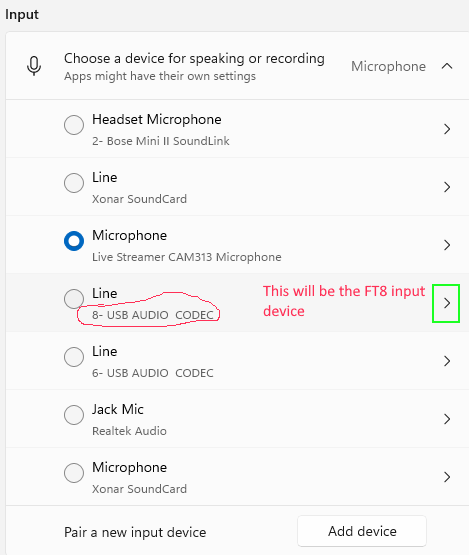In the depicted image, there is a user interface for selecting and configuring an audio input device. The upper left section of the image features a gray background, with the word "Input" written in either dark gray or black text. Below this, a white rectangular overlay contains additional settings.

On the left side of the overlay, there are icons for a speaker or microphone. To the right of these icons, instructions read: "Choose a device for speaking or recording." Beneath this text, in small gray font, it mentions that "Apps might have their own settings." 

Towards the far right, in gray text, the term "Microphone" is displayed alongside an upwards-pointing arrowhead, indicating an expandable menu below. The list of audio devices follows, each accompanied by respective tick boxes and arrowheads pointing to sub-menus:

1. **Headset Microphone**:
   - Beneath the bold black text of the device name, the words "Bose Mini 2 Sound Link" are written in gray, followed by a right-pointing arrowhead.

2. **Line**:
   - This option lists "Xonar Sound Card" in gray text with a corresponding right-pointing arrowhead.

3. **Microphone (Selected)**:
   - Enclosed in a thick blue border, indicating it is the active selection, this option reads "Microphone" in black text. Below it, in gray lettering, "Live Streamer CAM 313 Microphone" is displayed, with a right-pointing arrowhead.

4. **Line (Circled)**:
   - This option contains the text "USB Audio CODEC" beneath the bold label "Line." Highlighted with a thin red line encircling it, the adjacent note in red text states: "This will be the FT8 input device." The item has a right-pointing arrowhead and is further highlighted with a lime green rectangle.

5. **Line**:
   - Below it, the text "USB Audio CODEC" is again mentioned, with a number "6-" preceding it. This item also has an accompanying right-pointing arrowhead.

The overall interface presented in the image appears to be designed for detailed audio input configuration, clearly displaying the various available audio devices and providing user-friendly options for selection and customization.